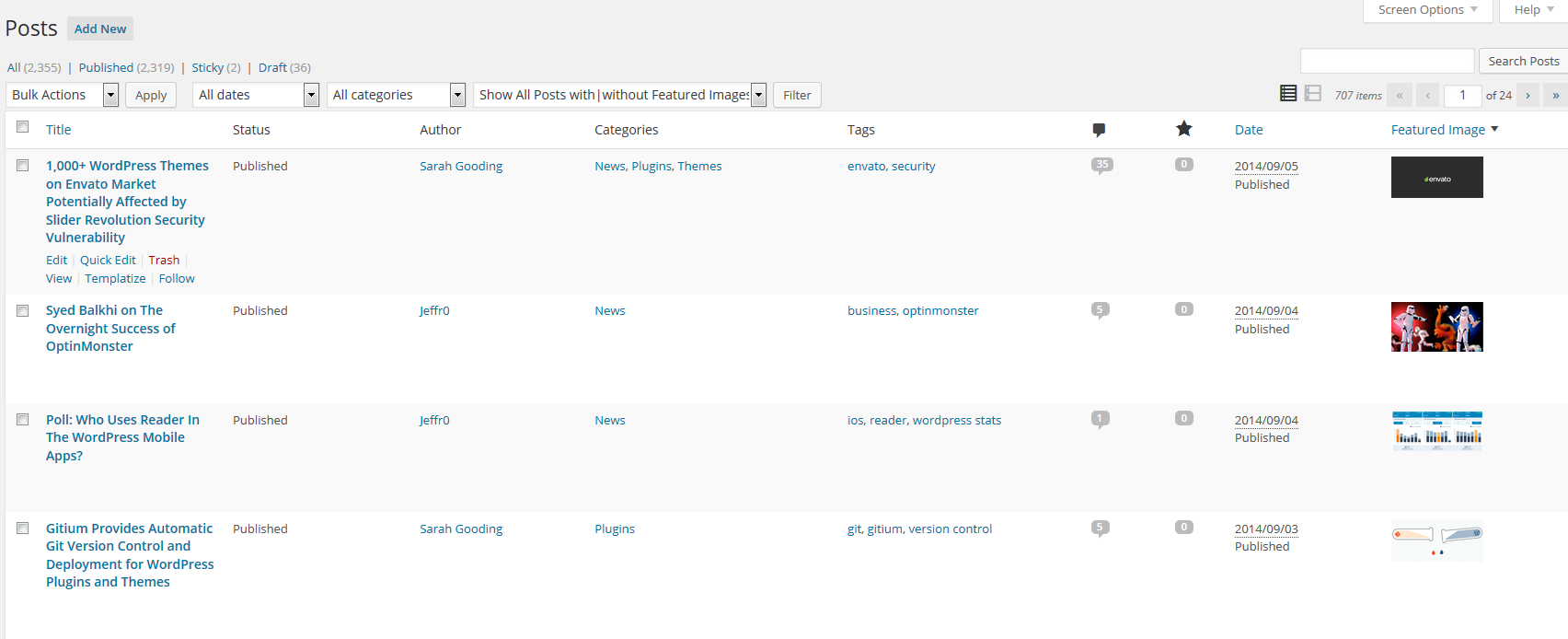This is a detailed screenshot of a blog management interface, likely from a content management system such as WordPress, displayed on a computer screen rather than a mobile device. The image has a landscape orientation, being wider than it is tall. At the top, a gray navigation bar is visible. On the upper left-hand corner of this bar, the word "Posts" is prominently displayed in black font. Adjacent to it, in a dark grey square, the option "Add New" is highlighted in blue font.

The interface indicates a total of 2,355 posts, with 2,319 published, 2 marked as sticky, and 36 in draft status – an extensive number for a single blog. Various actions can be performed via drop-down menus labeled "Bulk Actions," "Apply All Dates," "All Categories," and "Show All Posts Without Featured Image."

The screenshot also includes a grid listing the posts, structured by column headings such as Title, Status, Author, Categories, Tags, Number of Comments, Number of Favorites, Date, and Featured Image. By examining the dates, it is evident that this blog has posts dating back to 2014, indicating it has been active for nearly a decade. 

One of the top entries features a post titled "1,000+ WordPress Themes on Envato Market Potentially Affected by Slider Revolution Security Vulnerability," suggesting that the blog focuses on insider news related to WordPress themes and security updates.